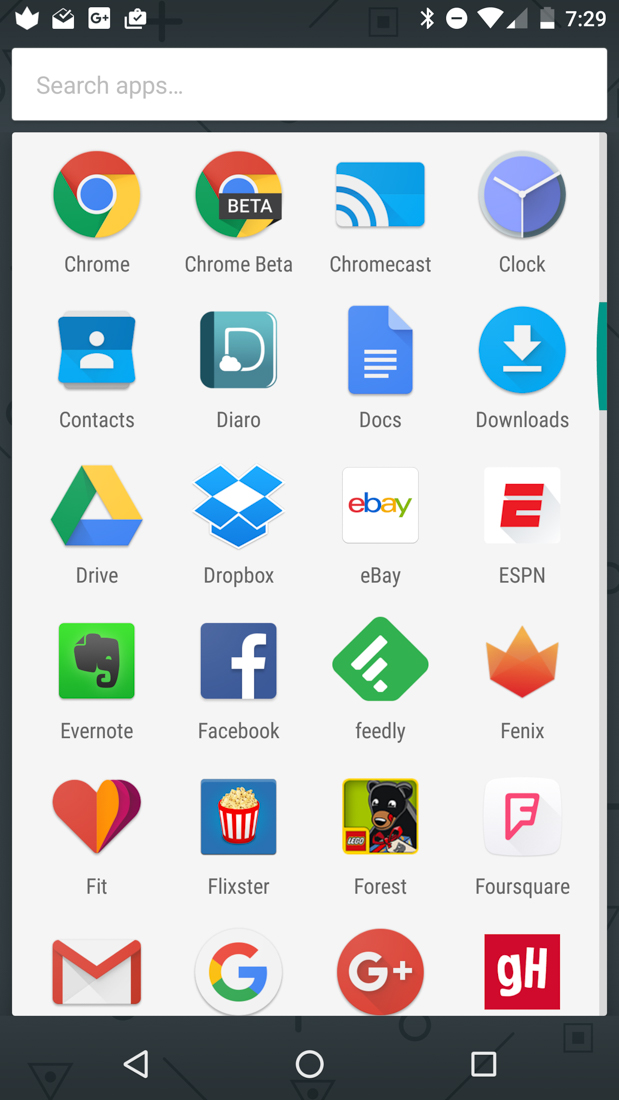This is a detailed smartphone screenshot showcasing the "Search Apps" page. At the top of the screen, there's a series of icons starting with a crown-like symbol, followed by a male user icon, a Google Plus icon, and a checked lock icon, indicating an active security feature. To the right of these icons is the Bluetooth logo, displayed within a white circle that contains a "minus" sign, a WiFi signal icon, and a battery indicator. The timestamp on the screen reads 7:29.

Below the icon row, there's a search bar labeled "Search apps," hinting at its function to find applications on the device. The main content displays a list of application icons in this order: Google Chrome, Chrome Beta, Chromecast, Clock, Contacts, Google Docs, Downloads, Drive, Dropbox, eBay, ESPN, Evernote, Facebook, Feedly, Phoenix (recognized as the symbol that was previously unknown), Fit, Flixster, Forest, Foursquare, Gmail, Google, Google Plus, and an app labeled GH.

Lastly, the bottom border of the screen is black with three navigational icons: a left-facing arrow (Back), a circle (Home button), and a square (Overview/Recent Apps button).